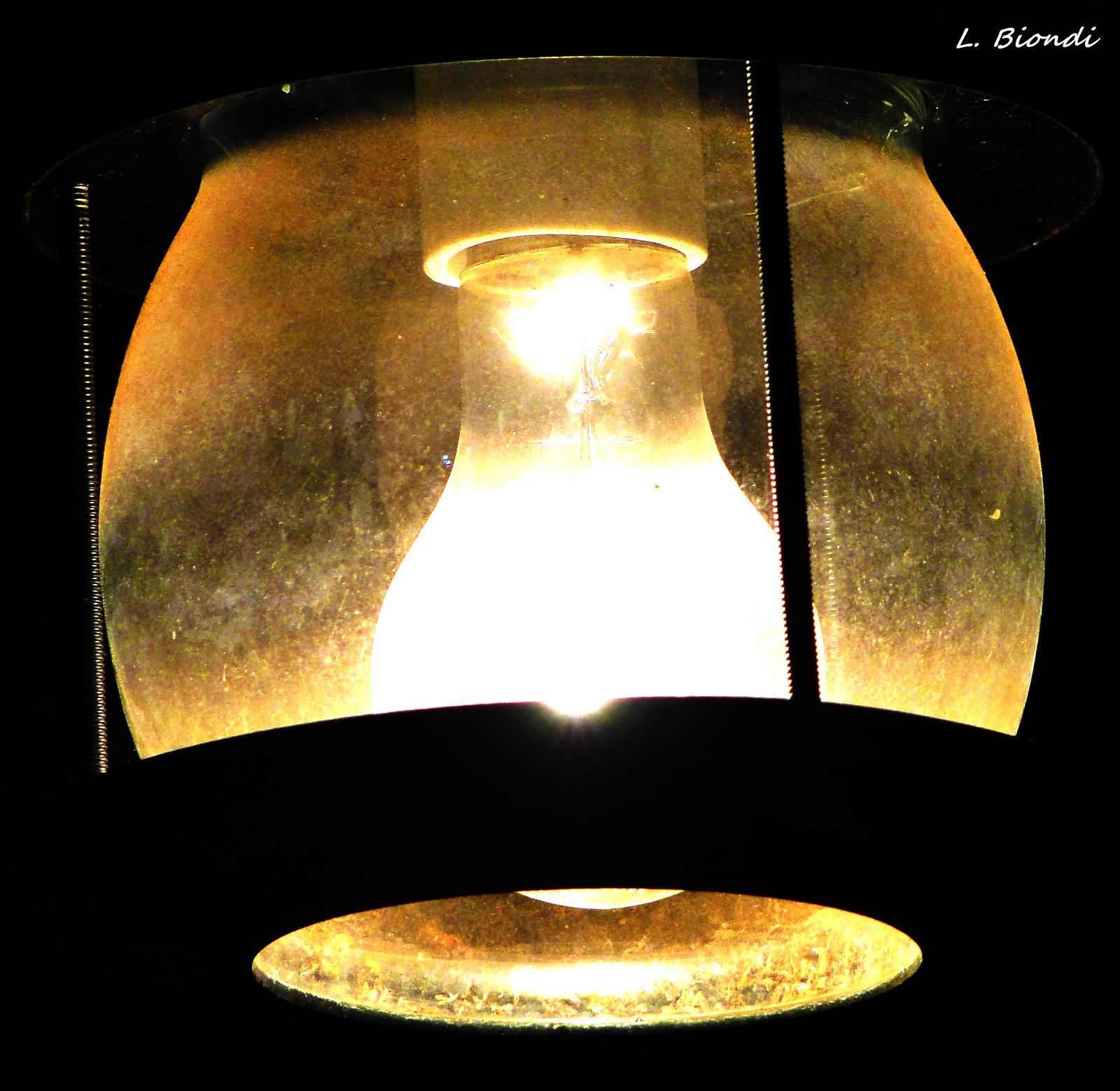The photograph depicts a close-up of a shining incandescent bulb housed within a lantern-like structure. The bulb emits a bright white light that casts an orange hue onto the surrounding glass dome. This glass dome appears yellowish due to the intensity of the light and is supported by a round, black metallic frame with long metal screws, giving the lantern stability and structure. The background of the image is pitch black, highlighting the glowing bulb’s luminescence. In the top right corner, there's the text "L.Biondi" written in white, possibly indicating the photographer's name.